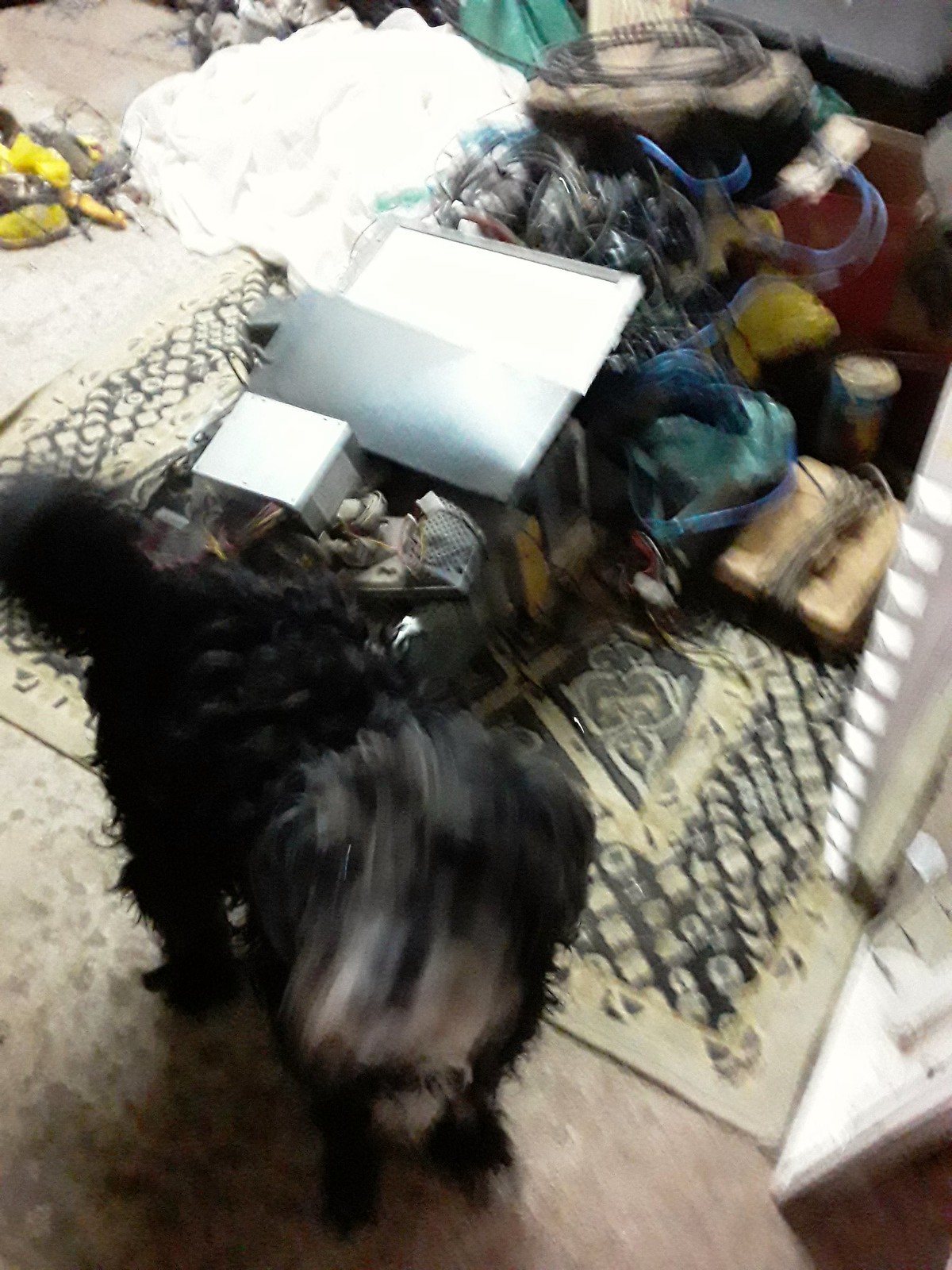This image, slightly rectangular and vertically oriented, captures a heavily blurred scene viewed from above. The photograph's top half reveals a chaotic assortment of variously colored objects—predominantly whites, blues, and a touch of red—scattered across an interior floor. The exact nature of these items remains indiscernible due to the significant blur. In the bottom half of the frame, amidst the visual haze, a dog looks up directly at the camera with an expression of curiosity. The dog’s snout is prominently whitish, contrasting with its predominantly black, curly fur covering the rest of its body. Despite the lack of clarity, the dog’s presence adds a notable point of interest to the otherwise confusing and cluttered scene.